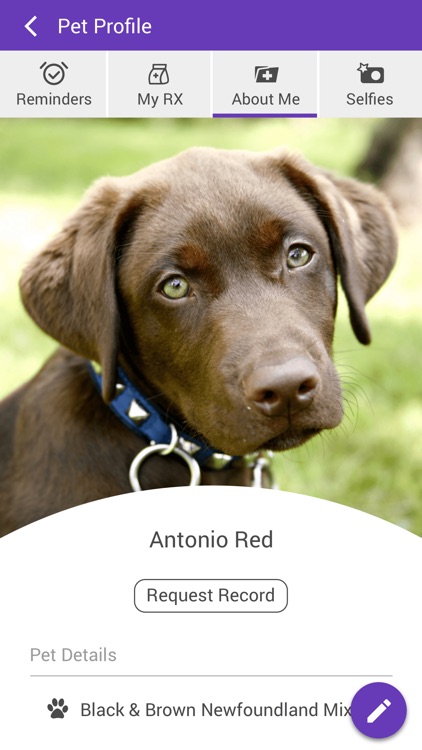The image shows a vertical screenshot of a website or app designed for pet care. At the top, a thin purple bar features the text "Pet Profile" in white, accompanied by a leftward arrow. Below that, four gray boxes, each separated by white lines, offer different options: "Reminders" with an alarm clock icon, "RX" with an icon of a bag and a plus sign, "About Me" underlined in purple with a folder and a plus sign, and "Selfies" with a camera and star icon.

Beneath these options, there's a photograph of a dog that appears to be a chocolate Labrador Retriever puppy. The puppy has striking green eyes, soft features, and light-colored whiskers. It is wearing a blue collar adorned with silver accents and two silver loops attached to additional loops on the collar. The background is slightly blurred, with hints of green grass and a tree in the top right corner, emphasizing the focus on the puppy's adorable face and droopy ears. 

Below the image, the text "Antonio Red" is displayed, followed by a "Request Record" button. Further down, there's a section labeled "Pet Details," featuring a paw print icon. It describes the dog as a "Black and Brown Newfoundland Mix." To the right of this description, a purple circle with a pencil icon signifies an option to edit the details.